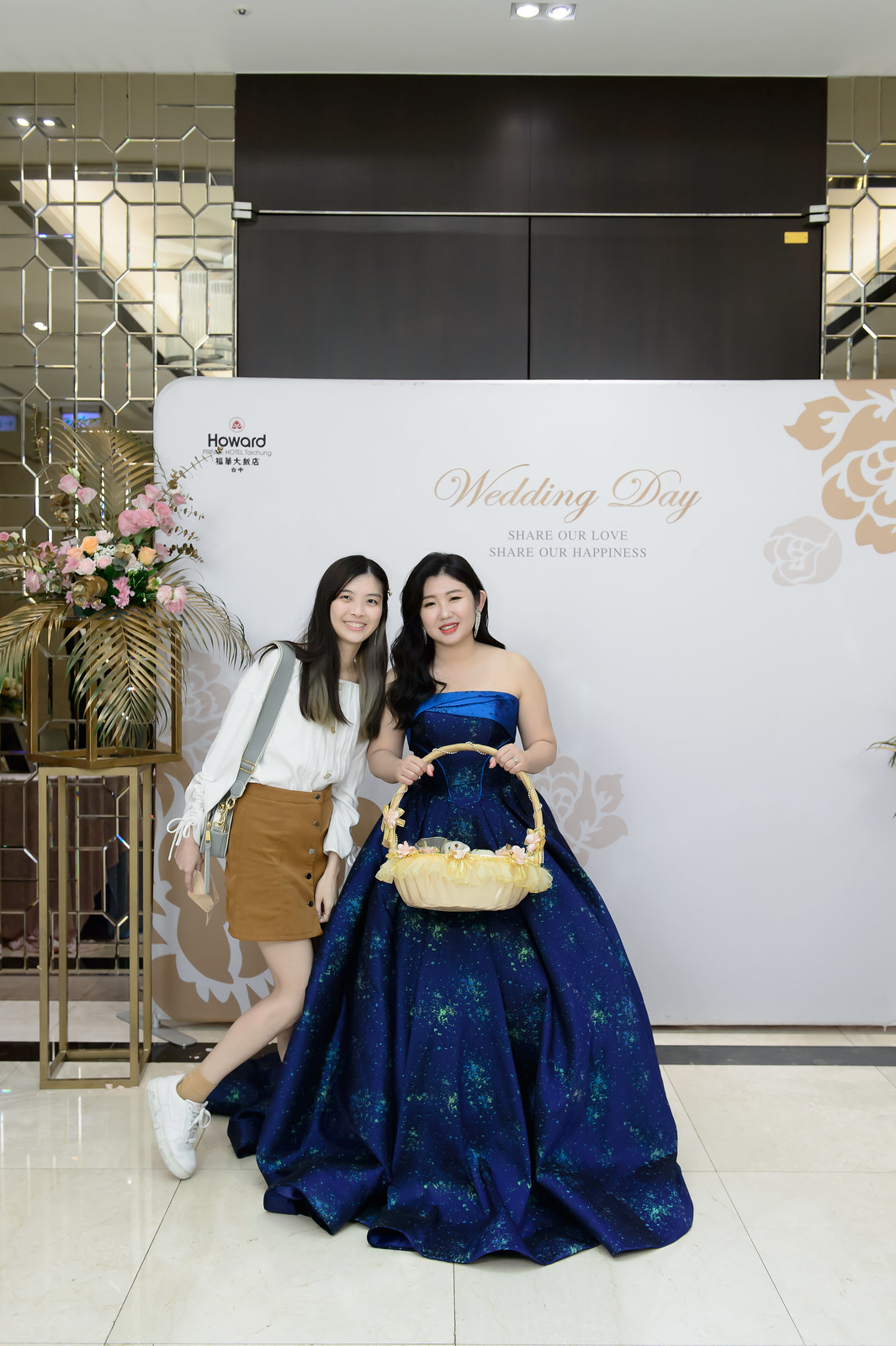In this photograph taken at the Howard Hotel in Taiwan, two women of Asian descent are posing in front of a minimalistic white panel adorned with illustrations of single-color flowers. The top part of the banner reads "Wedding Day. Share our love, share our happiness." On the right stands Elise, possibly the bride or a maiden of honor, dressed in a luxurious, long, dark blue gown with hints of neon green glitter. She holds a large beige basket full of flowers. The woman on the left, wearing a white long-sleeve button-up shirt, a brown skirt with buttons, white shoes, and tan socks, appears to be a guest or a friend posing with Elise. The scene exudes a joyful and celebratory atmosphere.